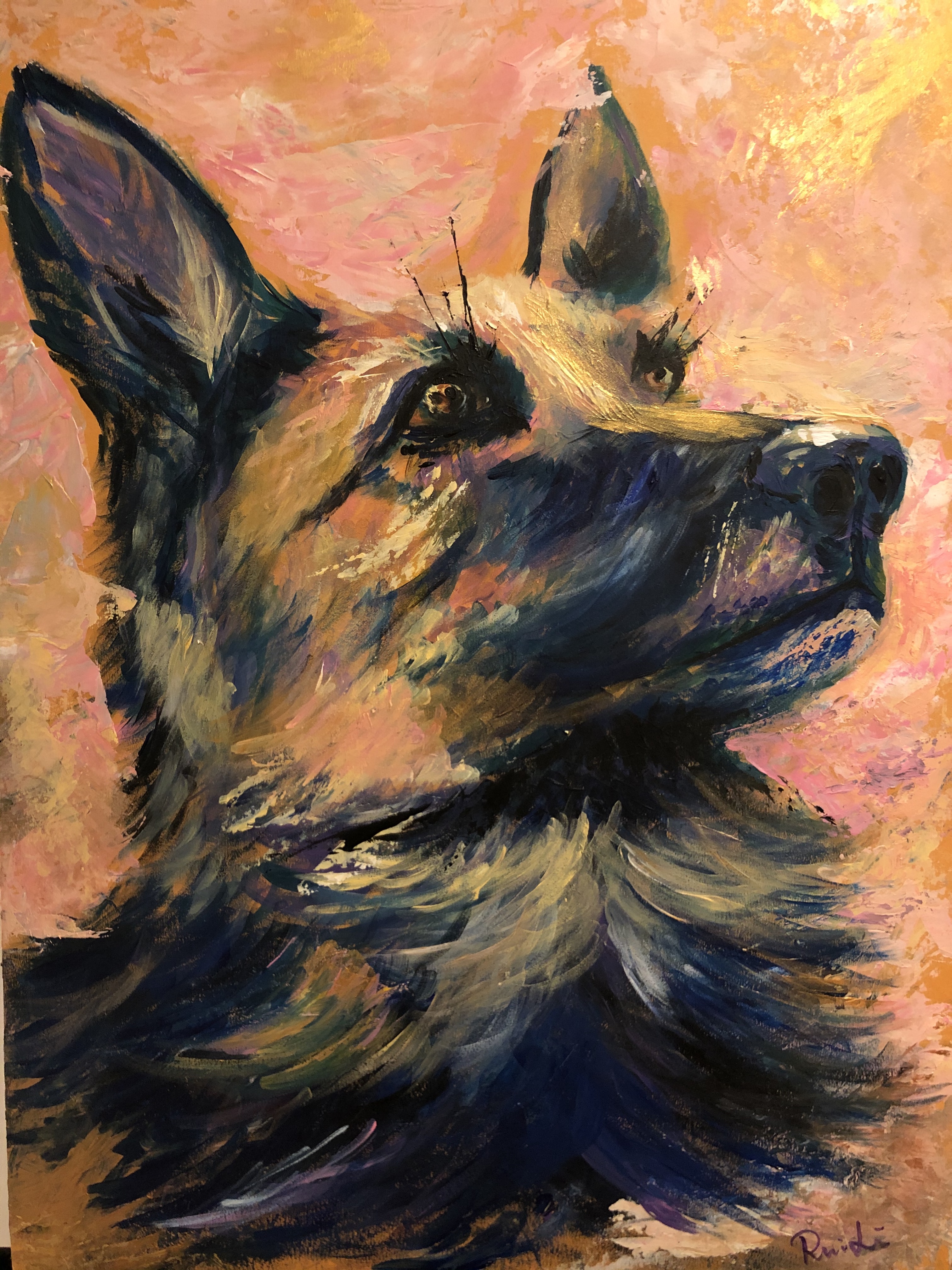This captivating oil painting masterfully captures the head and shoulders of a regally posed German Shepherd dog. The dog is portrayed with its mouth closed, pointy ears standing upright, and an expression of looking up and away towards the right. The artist employed large brushwork to create the realistic depiction of the dog's black and grey fur, with distinct orange markings around its eyes, a black nose, and touches of tan on the inner ears. The fur on the dog’s head is a blend of black, grey, and hints of tan and brown across its neck, evoking a sense of depth and texture.

The background is a vibrant array of colors: orange splashes interspersed with bold strokes of red, yellow, and grey, reminiscent of a sunset washing over the setting. This colorful backdrop contrasts beautifully with the dog's detailed, lifelike appearance, giving the painting a dynamic and lively atmosphere. The painting is signed by the artist as "RUIDI" in the bottom right corner, attesting to the creator's skill and attention to detail.